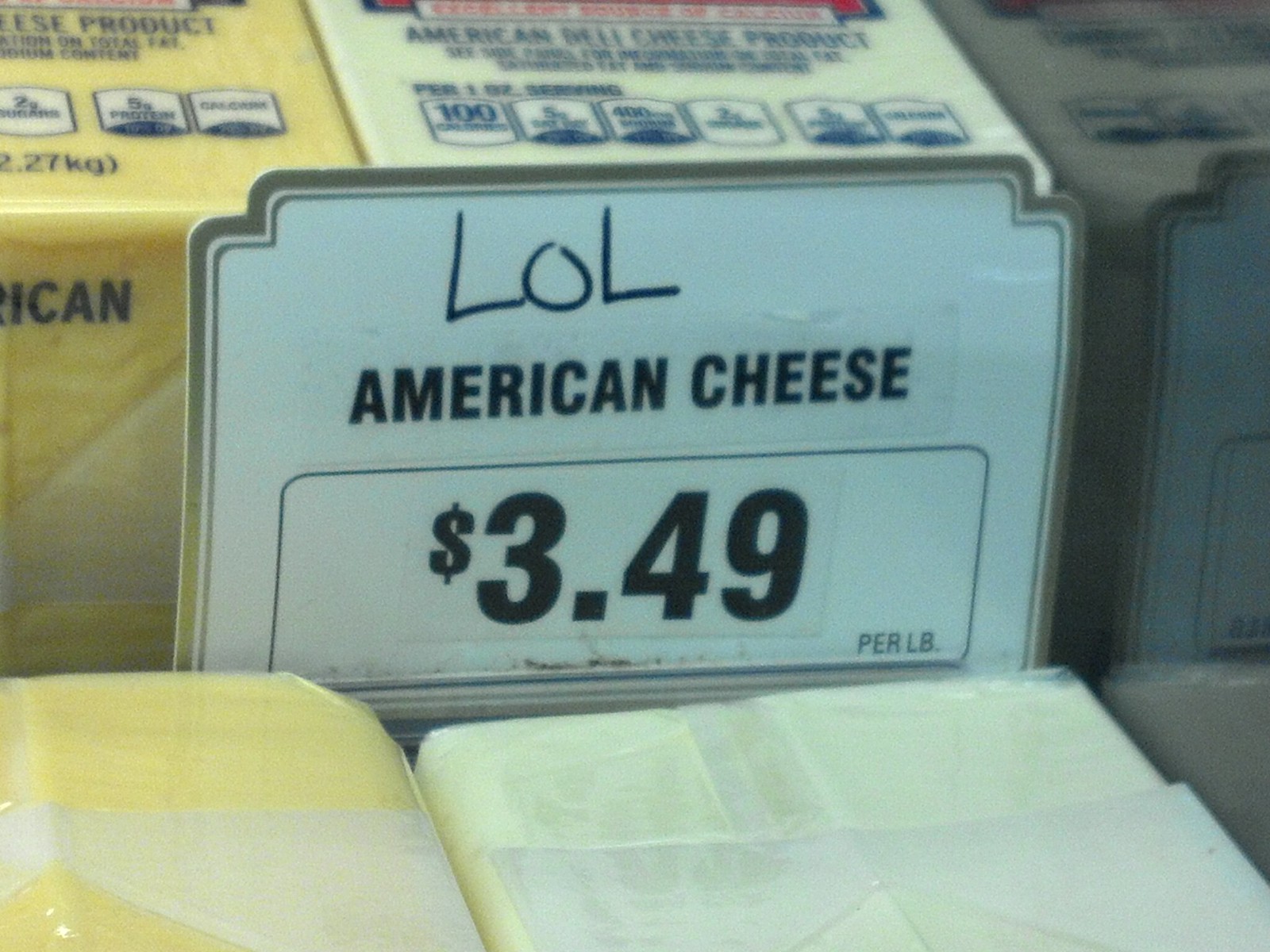This photograph prominently features a white sign with black, handwritten-style font, bordered in gray. The sign reads "LOL," followed by "AMERICAN CHEESE" in all capital letters. Below this text, a black rectangle highlights the price, which is listed as $3.49 per pound. In front of the sign, several pieces of plastic-wrapped cheese are visible, predominantly white with some showing a whiter orange hue. Behind the sign, there are larger cheese blocks with nutrition facts labels, also wrapped in plastic. The sign has a slight light reflection, contributing to the photograph's somewhat grainy appearance, suggesting that the image may be older. The overall scene appears to be a display of cheese products with a focus on American cheese.